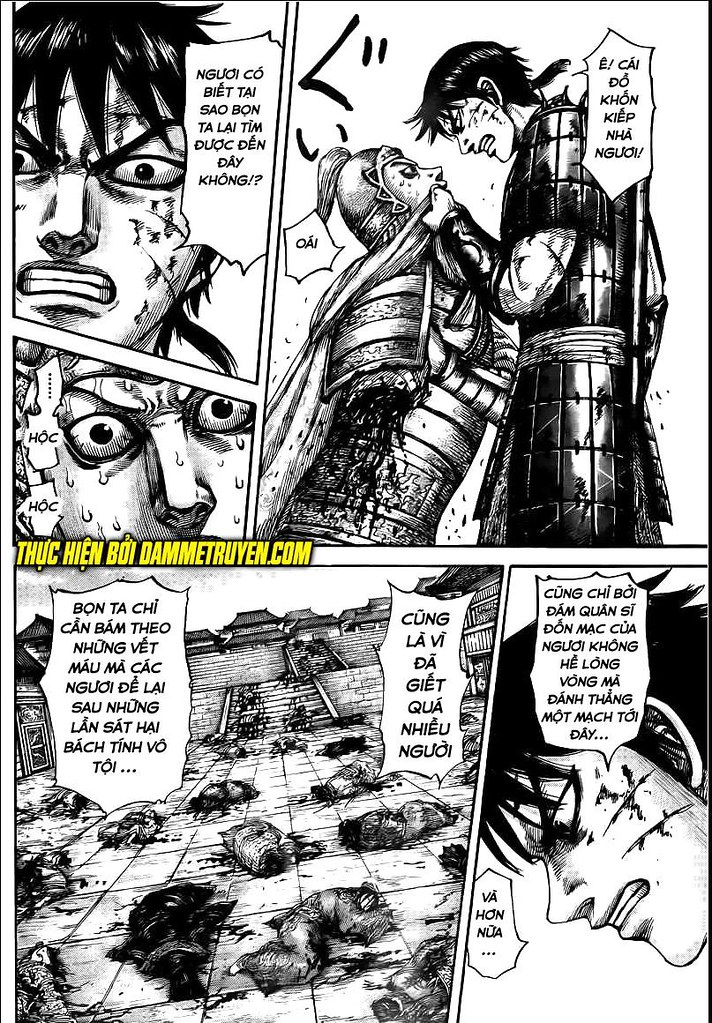This is an image of a manga comic book page presented in a vertical rectangular shape, showcasing detailed black and white artwork. The composition is divided into five panels: two on the top left, one large panel on the top right, a large panel on the bottom left, and a smaller panel on the bottom right. Each panel contains dialogue in an unreadable foreign language, possibly Vietnamese.

In the top left panel, an angry man with gritted teeth is depicted, with his face contorted in fury. Below, on the left, he is seen forcefully holding another man by the collar, who looks troubled and frightened. These characters are dressed in knight-like attire, suggesting a medieval or fantasy setting.

The large top right panel displays a striking scene of numerous dead bodies strewn across what appears to be an ancient, grandiose structure, reminiscent of an old Chinese emperor's temple or a massive concrete arena. This setting is rich with an Asian architectural aesthetic, evoking a historical ambiance.

In the smaller bottom right panel, the angry man from earlier is shown again, looking down as he speaks to an unseen person. The overall atmosphere is tense and action-packed, contributing to the dramatic tone of the narrative. The page is predominantly monochromatic, with the exception of some overlaid yellow text on the middle left panel, which reads "tokienboydamitryen.com," suggesting an added annotation or watermark.